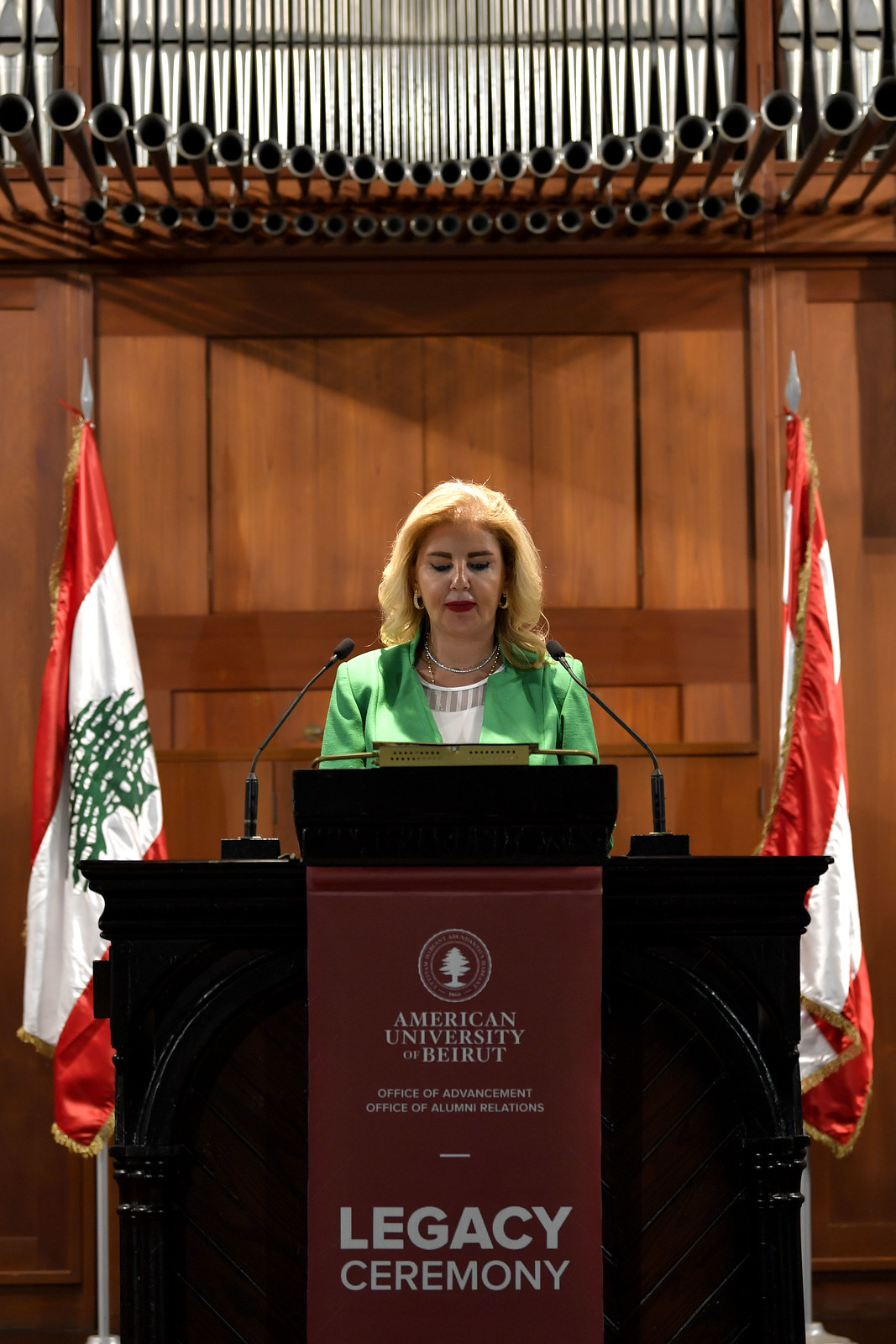This detailed color photograph features an attractive middle-aged, fair-skinned woman standing behind a black podium adorned with a maroon banner that reads "American University of Beirut Office of Advancement, Office of Alumni Relations. Legacy Ceremony" in white letters. The woman, who appears to be in her 50s, has shoulder-length blonde hair and is elegantly dressed in a bright green blazer over a white shirt with fringe around the collar. She is accessorized with diamond hoop earrings, a diamond necklace, a pearl necklace, and red lipstick. Situated behind her is a dark wooden wall, likely part of a pipe organ, with metal tubes and horn-like ends visible at the top of the image. Flanking her on both sides are two vertical red and white striped flags, with one flag showing a partial green symbol. The woman looks down, seemingly reading from her notes, with two microphones positioned at either side of her head.